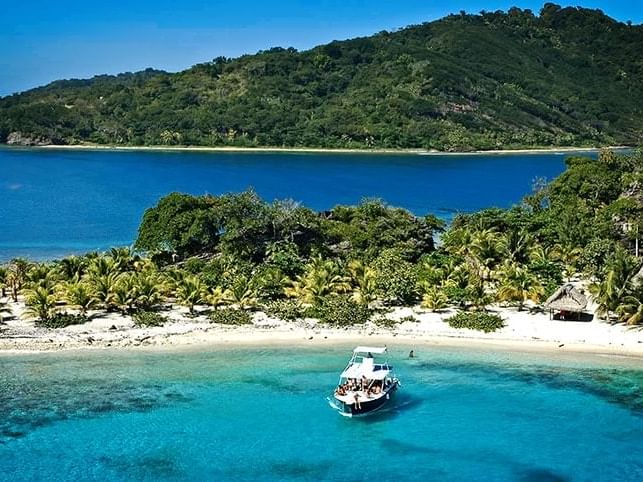This vibrant, aerial photograph captures a tropical paradise with stunning detail. The image showcases a small, lush island with light-colored sand and dense greenery, including numerous palm trees. Centered in the frame is a white motorboat with an awning, appearing to be a touring vessel filled with people enjoying their day. The boat sails in the lighter, teal-blue section of the water, which contrasts beautifully with the darker, deeper blue hues of the adjacent sea. The island boasts a quaint thatched-roof hut nestled among the trees. In the background, another, larger island rises with steep, jungle-like terrain, adorned with more trees and a thin stretch of beach. The clear blue sky overhead enhances the serene and picturesque quality of this tropical scene.